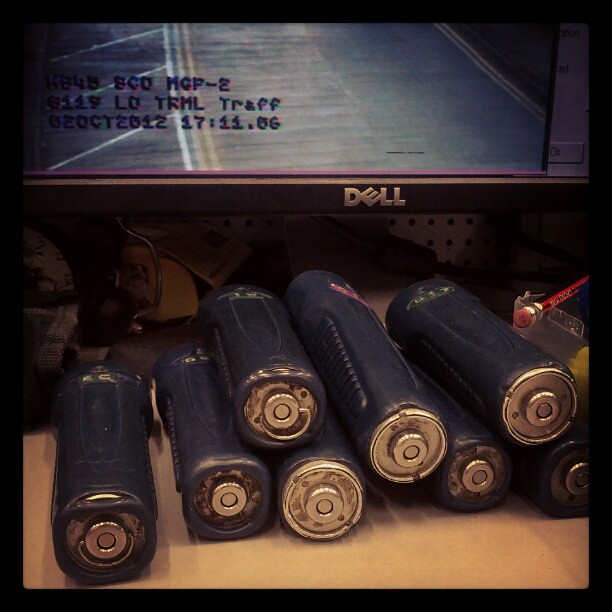The image depicts a detailed scene from what appears to be an indoor workshop environment, with a Dell computer monitor prominently positioned towards the back. The lit-up monitor screen displays footage of an empty roadway, marked with various alphanumeric codes including "KB45BCOMGP-2," "119LDTRMLTRAFF," and "620CT2012 at 71106." In front of the monitor, set on a workbench or tabletop, are eight blue rubber-wrapped objects resembling batteries or flashlights, each with silver metal caps, some appearing corroded. These items are arranged in a slightly disorganized manner, potentially even in a pyramid-like fashion. Also present on the tabletop is a red pencil with an eraser and a gold tip, propped against the blue objects. The background suggests a workshop setting, possibly a basement, indicated by the pegboard with hooks on the wall, adding to the eclectic assortment of items.